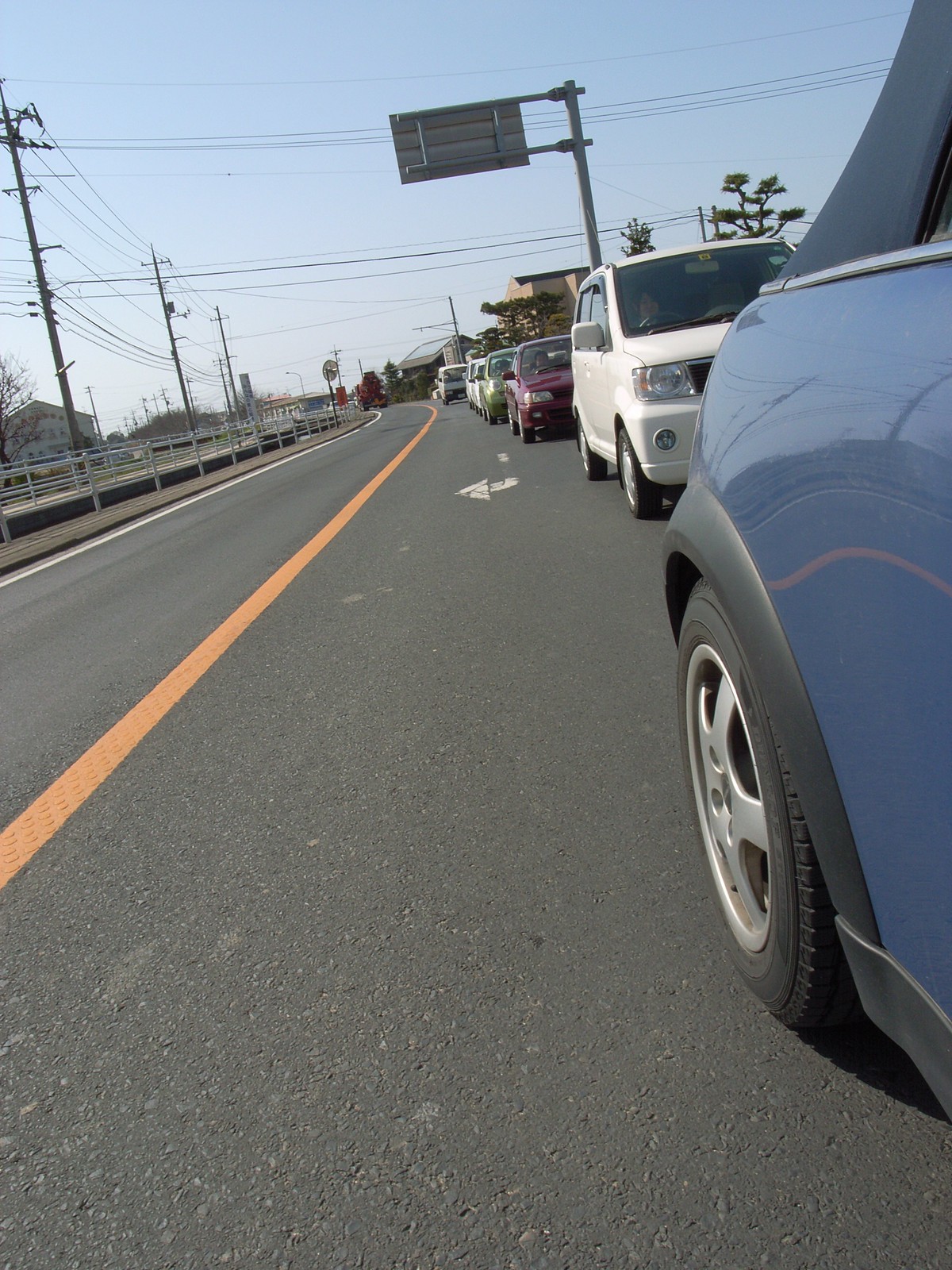A photograph taken from the middle of a two-lane road captures a bright, sunny day with clear blue skies. The perspective looks backward, revealing a queue of five to six cars in various colors, including white, purple, and green, trailing behind. Each car has passengers visible, waiting patiently. The road, defined by a yellow line running down the center, is bordered by houses in the distance, adding a suburban touch. Electrical pylons line the road’s edge, contributing to the elements of everyday life captured in this vibrant and busy scene.